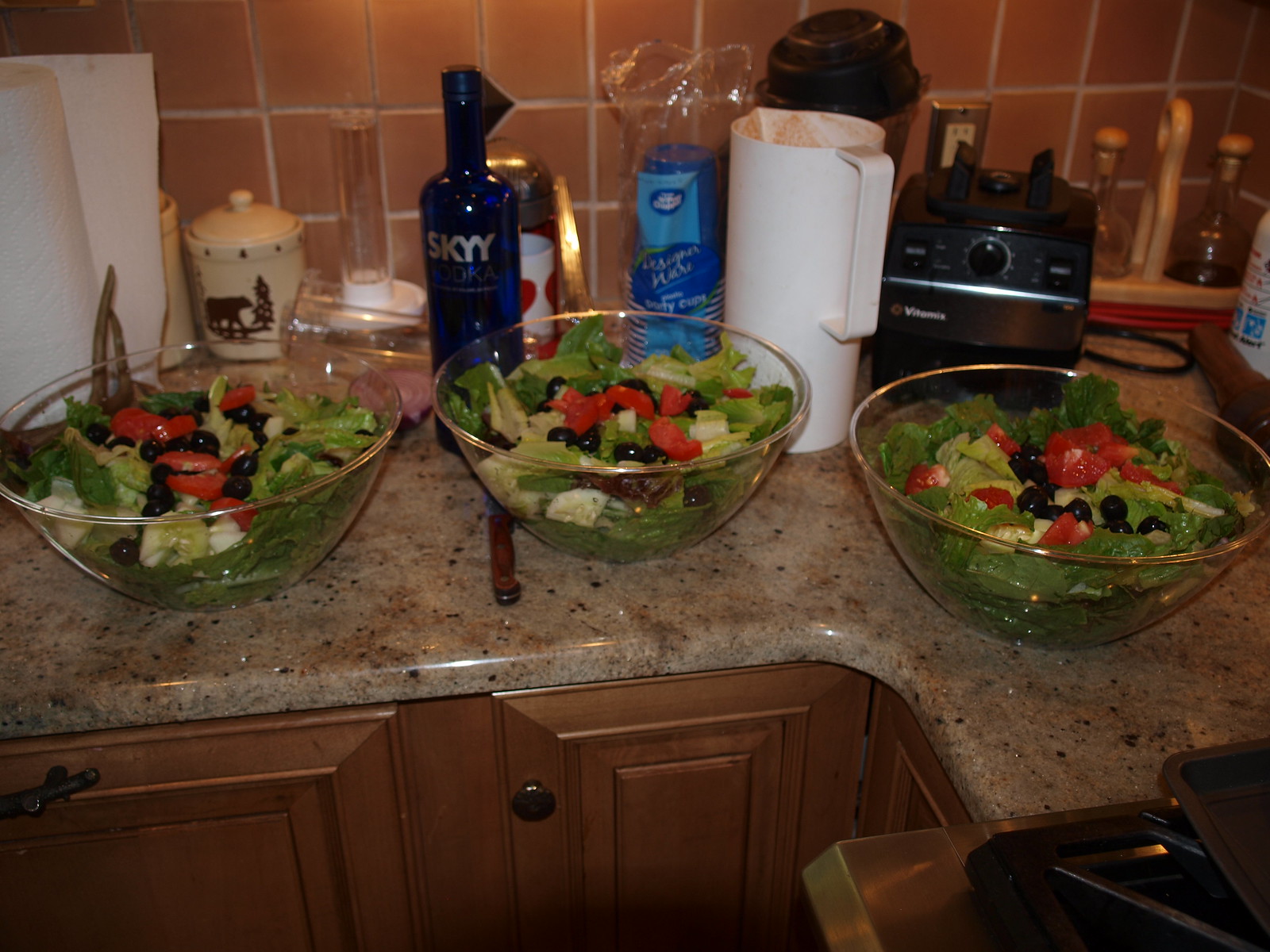This detailed photograph captures a cozy corner of a modern kitchen. At the forefront, a sleek granite countertop, rounded at the corner, sets the stage with its grayish, marble-like finish. Below the countertop, stylish blonde wood cabinets with metal handles add warmth and contrast. The centerpiece of the image is four large bowls brimming with garden salads. Each bowl is teeming with fresh green lettuce, vibrant red tomatoes or peppers, and dark olives or grapes, creating a colorful feast for the eyes. Among the salads, a striking blue SKYY Vodka bottle stands out, flanked by a white pitcher and a blender base with its plug visible. The background reveals a brick wall with white-lined squares, adding a rustic element to the scene. Additional kitchen accessories, including a white paper towel roll and a sugar jar, complete the inviting kitchen atmosphere.